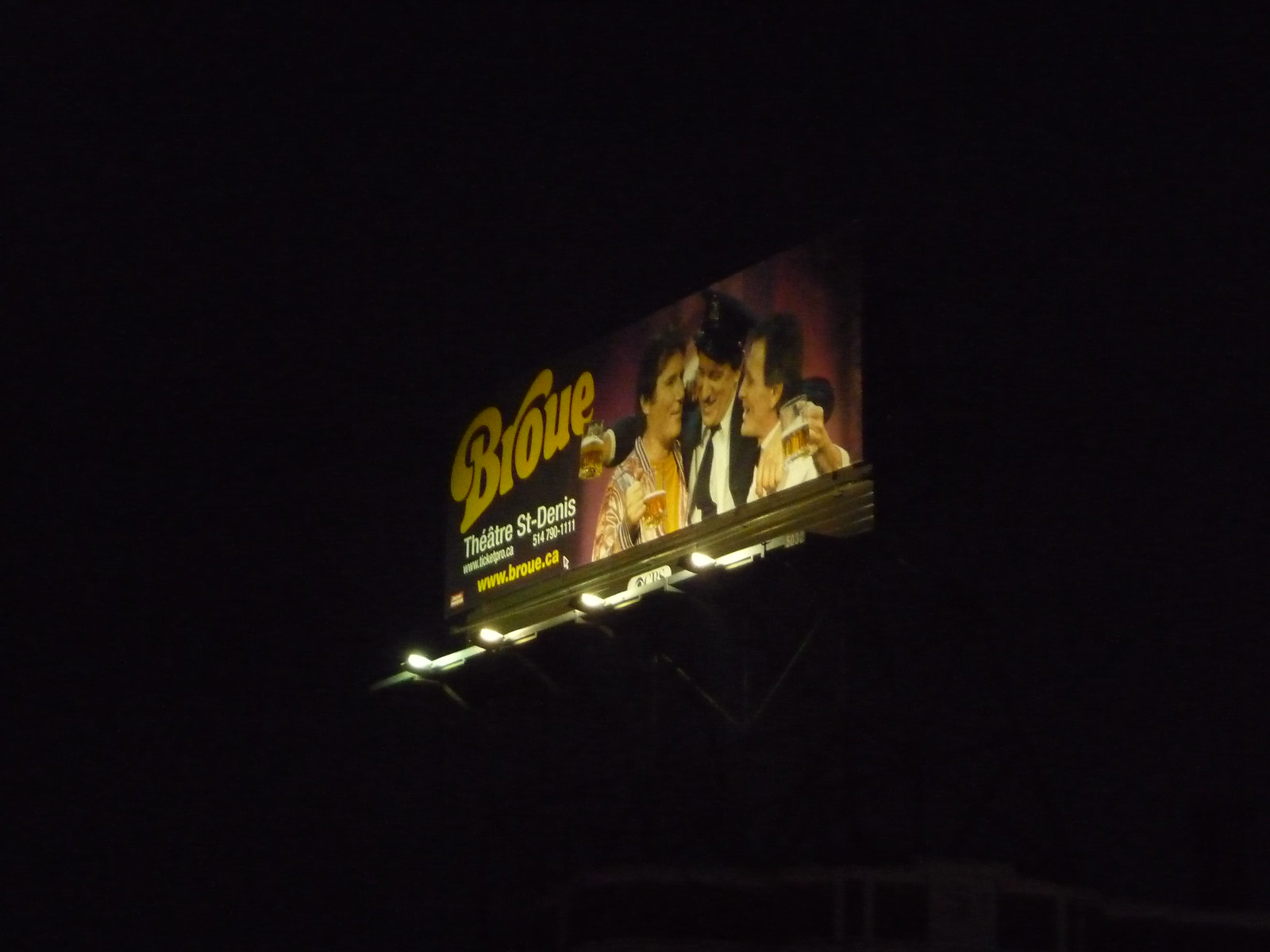This photograph captures a billboard against a pitch-black night sky, creating a striking contrast that draws all attention to the well-lit sign. The billboard, situated slightly above a barely discernible structure in the bottom right, is illuminated by four upward-facing lights at its base. Dominating the left side of the billboard are the bold letters "B-R-O-U-E," beneath which additional text appears, including "Theater St. Denis," a phone number ending in "1111," and the website "www.broue.ca." Centrally featured on the right side of the billboard is an image of three men in a celebratory pose. One man, distinguished by a hat that resembles either a chauffeur's or a policeman's hat, has his arms wrapped around the shoulders of the other two men. Each of the men is holding a glass mug, presumably filled with beer, enhancing the sense of camaraderie and festivity. The key visual elements—the dark night, the illuminated billboard, the website "broue.ca," and the trio of men in mid-celebration—come together to suggest a vibrant theatrical performance or advertisement related to a popular beer-themed show or event.